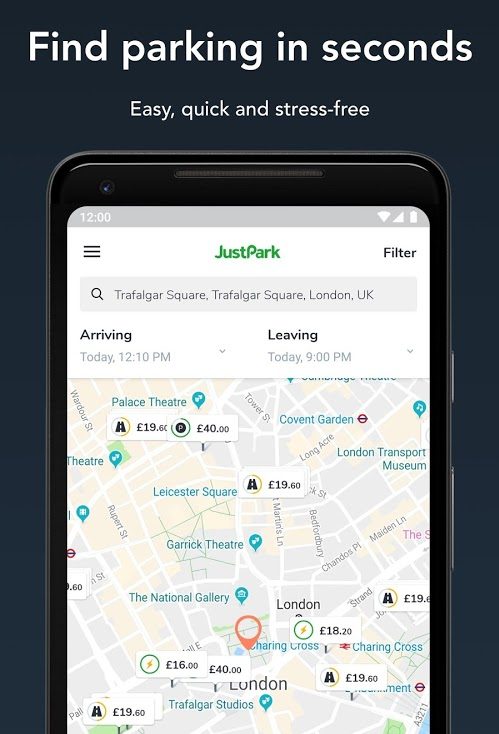**Caption:**

On a sleek black background, bold white letters at the top state, "Find parking in seconds, easy, quick, and stress-free." Below, an image of a smartphone is prominently displayed, focusing on the screen. It's 12:00 PM as indicated by the top of the screen. To the left, a hamburger menu icon is visible. Central to the screen, the app title "Just Park" is highlighted in blue and green. On the right, there's a "Filter" option. Directly beneath, a search box shows the location "Chappagall Square, London, UK." Further down, details of the parking session read "Arriving today 12:10 PM" and "Leaving today 9:00 PM." The bottom half of the screen displays a map of a section of London, pinpointing various notable locations such as the Palace Theatre, Leicester Square, Garrett Theatre, the National Gallery, Chappagall Studios, Charing Cross, Covent Garden, the London Transport Museum, and Charing Cross.